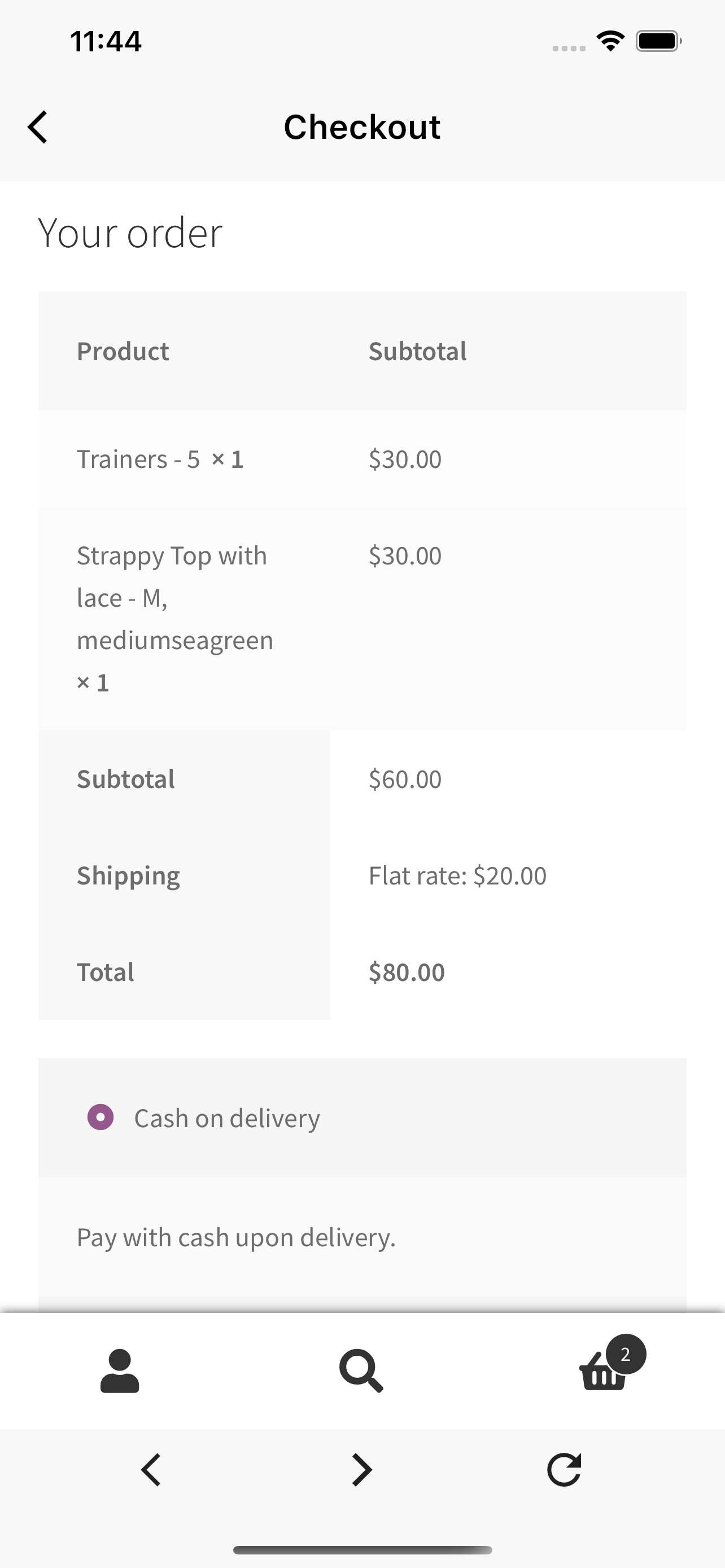This image is a screenshot taken from a mobile device, displaying a checkout page from a website or app. At the very top, there's a horizontally-aligned gray banner. On the left side of this banner, the time is displayed as 11:44, while the right side features icons indicating cellular signal strength and battery level.

Below the banner, aligned to the left, there's a left-facing arrowhead followed by the page title, "Checkout." Directly underneath, the heading "Your Order" is shown. The order summary begins with "Product Trainers, 5X1, subtotal $30," followed by "Strappy Top with Lace, M, Medium, Sea Green, X1, $30." The subtotal for both items is displayed as $60, with an additional flat-rate shipping fee of $20, bringing the total to $80.

Further down, there is a small round purple icon with an empty center, accompanied by the text "Cash on Delivery," which indicates that payment can be made in cash upon delivery of the items.

At the bottom of the screenshot, there is a row featuring three icons: a profile icon depicting a silhouette of a person on the left, a magnifying glass in the center, and a shopping cart icon on the right.